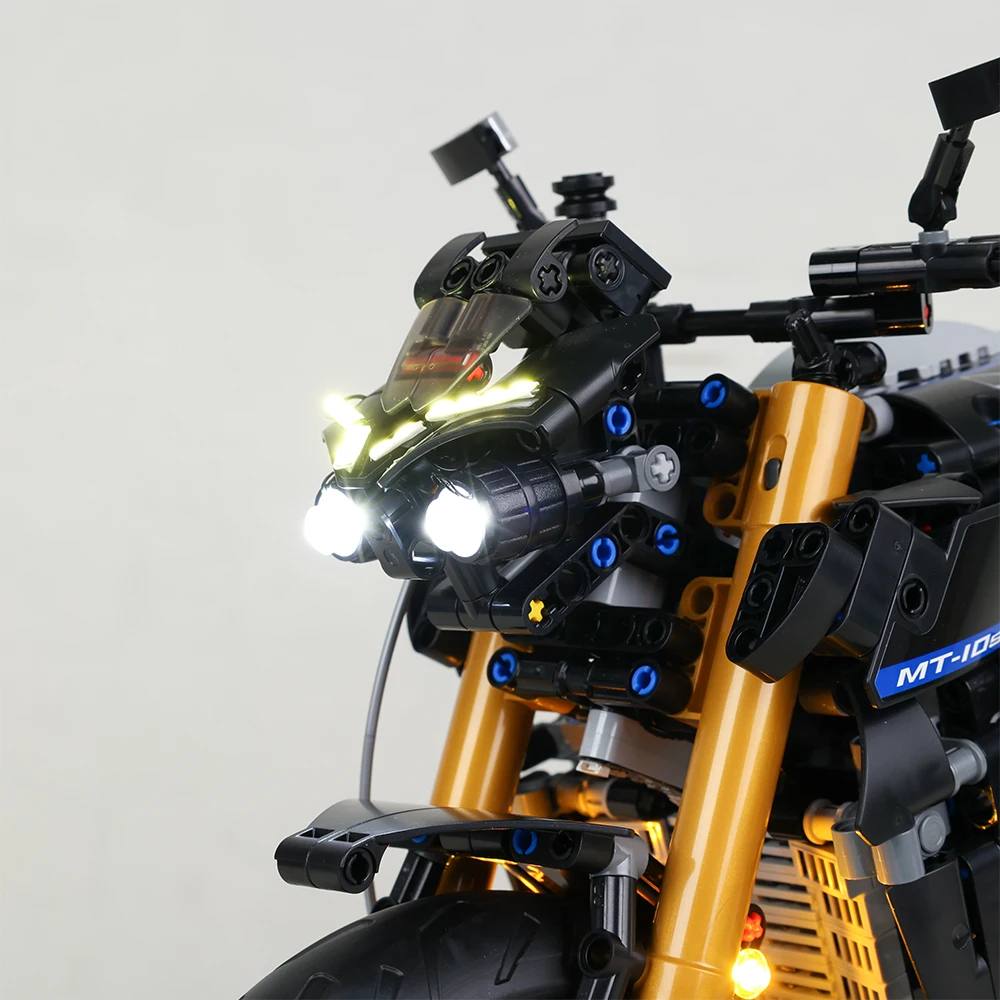The image depicts a close-up view of the front end of a futuristic, toy-like motorcycle with a gray background. The motorcycle exhibits a sleek and shiny design, reminiscent of a high-end Lego creation. The front showcases a pair of distinctive, individual headlights resembling eyes, giving the appearance of a face. The motorcycle's base is primarily black, with prominent yellow-gold bars on either side of the tire, which showcases traditional ridges. These bars seem to connect to the wheel, adding to the bike's structured design. The handlebars, which could also be mirrors, extend outward with a detailed finish. Bright blue screws are visible at the front, adding a pop of color against the darker tones and further emphasizing the intricate assembly. The front appears to lack a covering plate, exposing the inner workings more than a typical motorcycle. Additionally, there's an orange-copper pipework element that adds to the motorcycle's sophisticated yet toy-like appearance. The material and build suggest a plasticky, articulate toy rather than a traditional metal motorcycle.